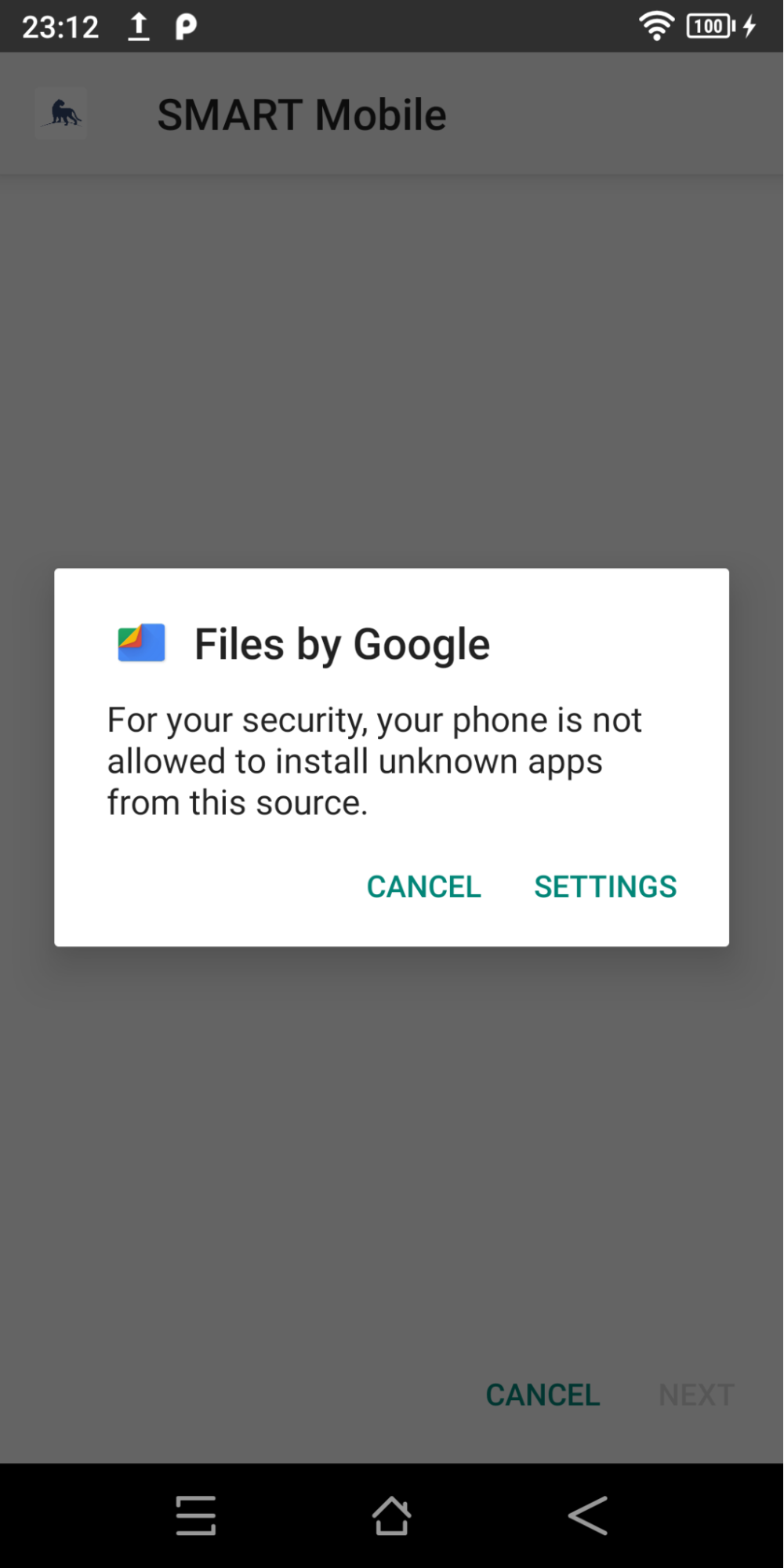The image shows a smartphone screen with the current time displayed as 23:12. The device is fully charged at 100% and is currently plugged in for charging.

At the center of the screen, a white pop-up from "Files by Google" is prominently displayed. Within this pop-up, a blue icon appears, although its exact design is indiscernible. The notification underneath the icon reads: "For security, your phone is not allowed to install unknown apps from this source." Options to either "Cancel" or access "Settings" are placed at the bottom of this notification, with the "Settings" option highlighted in green.

In the background, the home screen is visible. At the top, the smartphone brand is displayed as "SMART Mobile," where "SMART" is fully capitalized and "Mobile" has a capital 'M' only. To the right of this text, an icon resembling a black cougar is present, inside a white box. Below this, a faint horizontal line stretches across the screen. 

At the bottom of the screen, the navigation bar contains a central home button, a leftward arrow on the left, and three horizontal lines on the right.